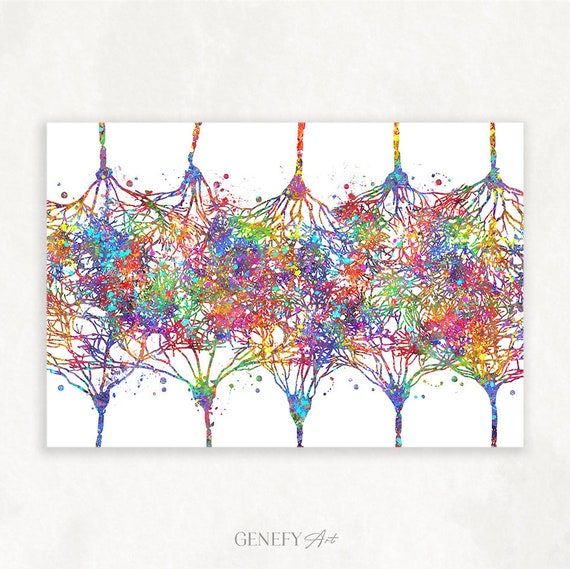This is a highly detailed, abstract painting by Genefy Art, displayed on an off-white, horizontal board. The overall composition of the image is square, without any borders, featuring a dominant off-white background. Central to the artwork are ten intricate, multi-colored root or string-like structures – five descending from the top and five ascending from the bottom. Each structure begins as a thin strip that branches out into a complex network of intertwining, vibrant roots or strings, creating tree-like forms with colored bulbs where they meet and intermingle. These roots showcase a kaleidoscope of colors including light blue, blue, violet, purple, red, orange, yellow, green, and aquamarine, with some areas displaying dots of color scattered around the bulbs. At the very bottom of the painting, centered, the artist's name "Genefy Art" is inscribed in gray. The repeated patterns and flowing color transitions give rise to a dynamic and visually engaging piece.